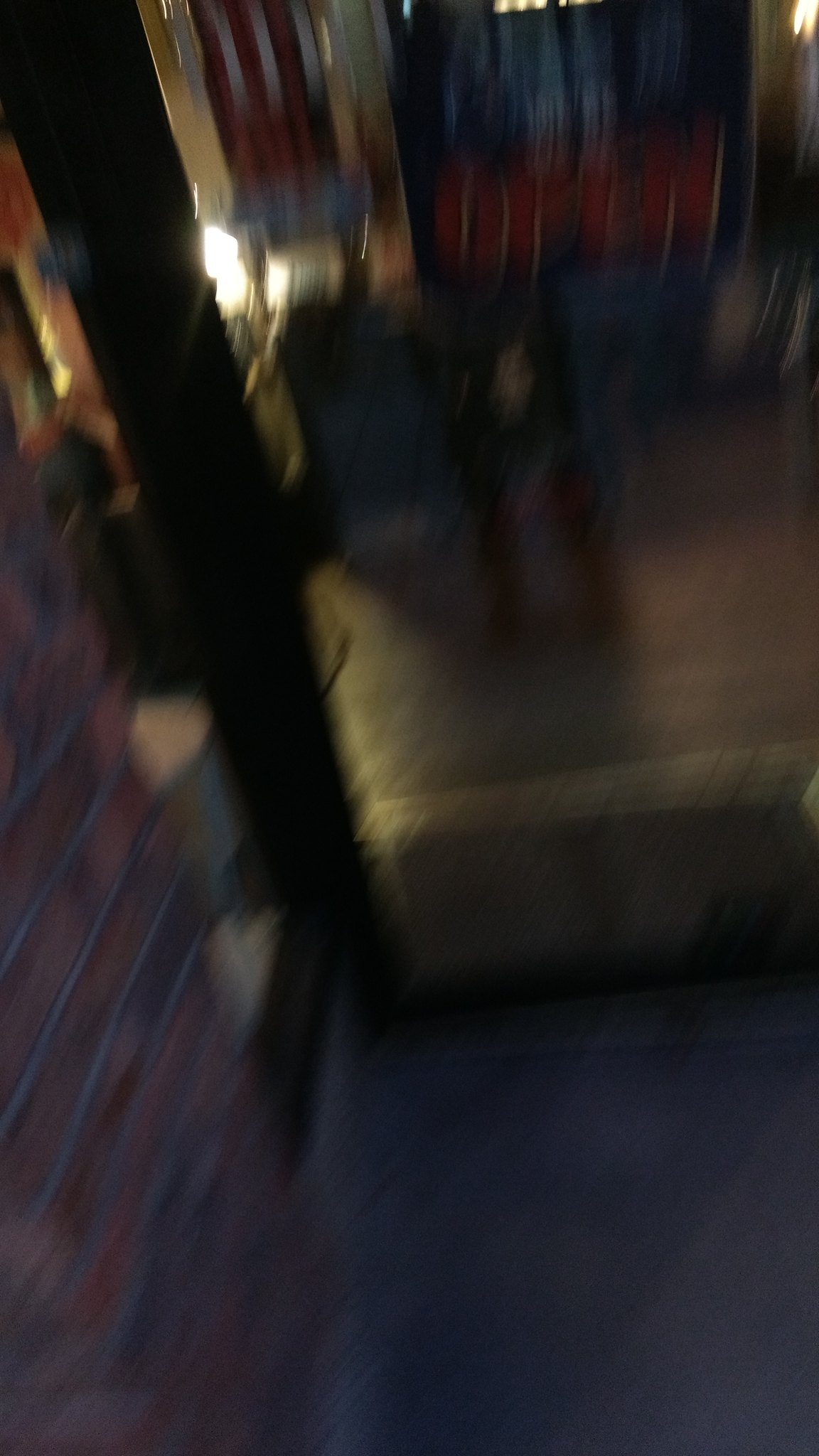In this extremely blurry image, the left-hand side features a brick wall adjacent to a dark wooden beam, which connects to the wall via a smaller beam near the floor. The floor appears to be made of gray concrete, leading up to a sizable step. In the background, there is a large, dark brown animal resembling a dog, standing on all fours. Behind the animal, bluish and reddish curtains are partially drawn, allowing sunlight to cast noticeable shadows. Two illuminated lights are visible, and around the corner, there's a faint outline of a mat or carpet. Despite the blurriness, the details offer a glimpse into a dimly lit, sunlit space with a mix of natural and artificial lighting.